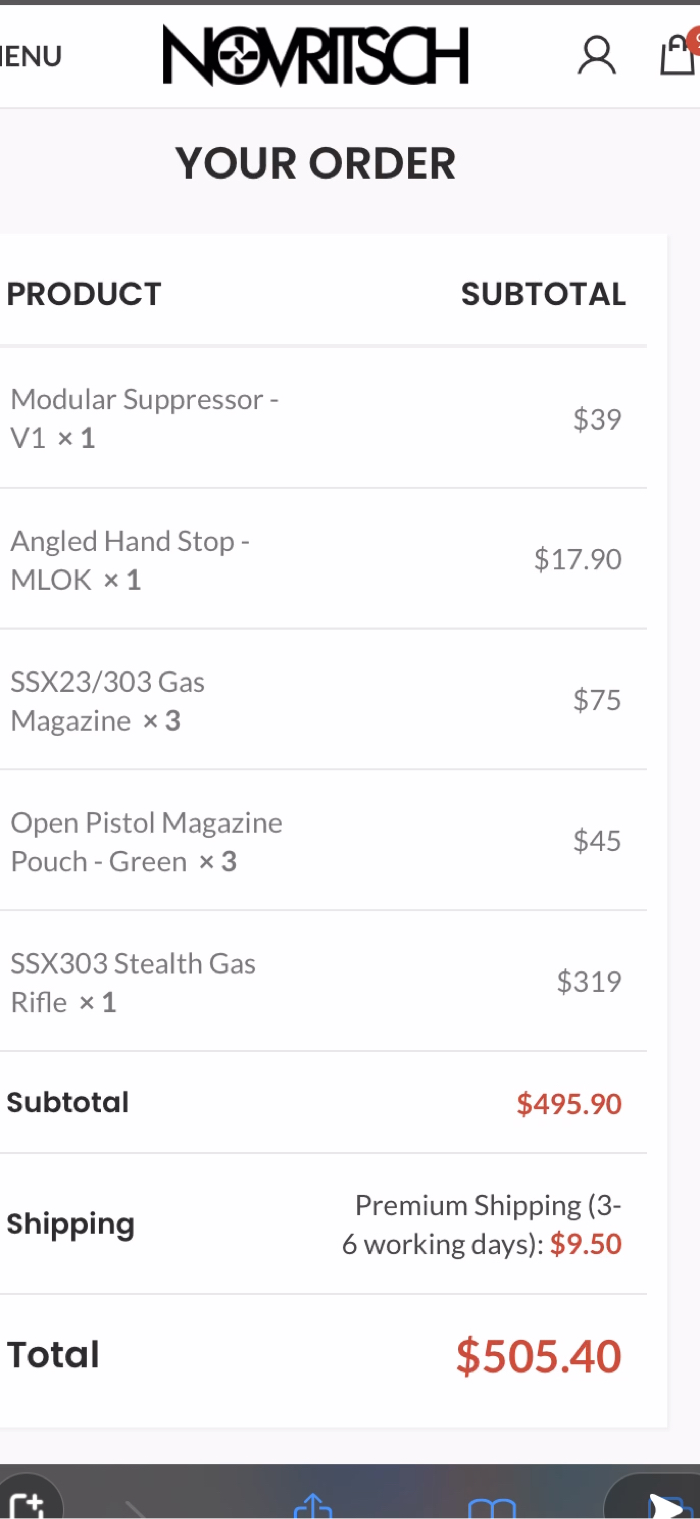This is a detailed screenshot from a mobile shopping cart on the Novritsch website. At the top center, the company's logo, "Novritsch," is displayed in black font, with a unique cross symbol embedded within the letter "O." To the left, the word "Menu" is partially visible with the "M" cut off. On the right, there are icons for the user account and a shopping bag.

Beneath the logo, the text "Your Order" is shown in a smaller font. Below this, a table is divided into two columns titled "Product" and "Subtotal." The "Product" column lists the items in the cart:
1. Modular Suppressor V1 x 1
2. Angled Hand Stop - MLOK x 1
3. SSX23/303 Gas Magazine x 3
4. Open Pistol Magazine Pouch - Green x 3
5. SSX303 Stealth Gas Rifle x 1

In the "Subtotal" column corresponding to each product, the prices are as follows:
1. $39
2. $17.90
3. $75
4. $45
5. $319

At the bottom of the product list, the subtotal of $495.90 is displayed, followed by the shipping cost of $9.50 for "Premium Shipping (3-6 Working Days)," resulting in a total cost of $505.40.

At the very bottom, a blue strip includes various phone-related functionalities for further actions.